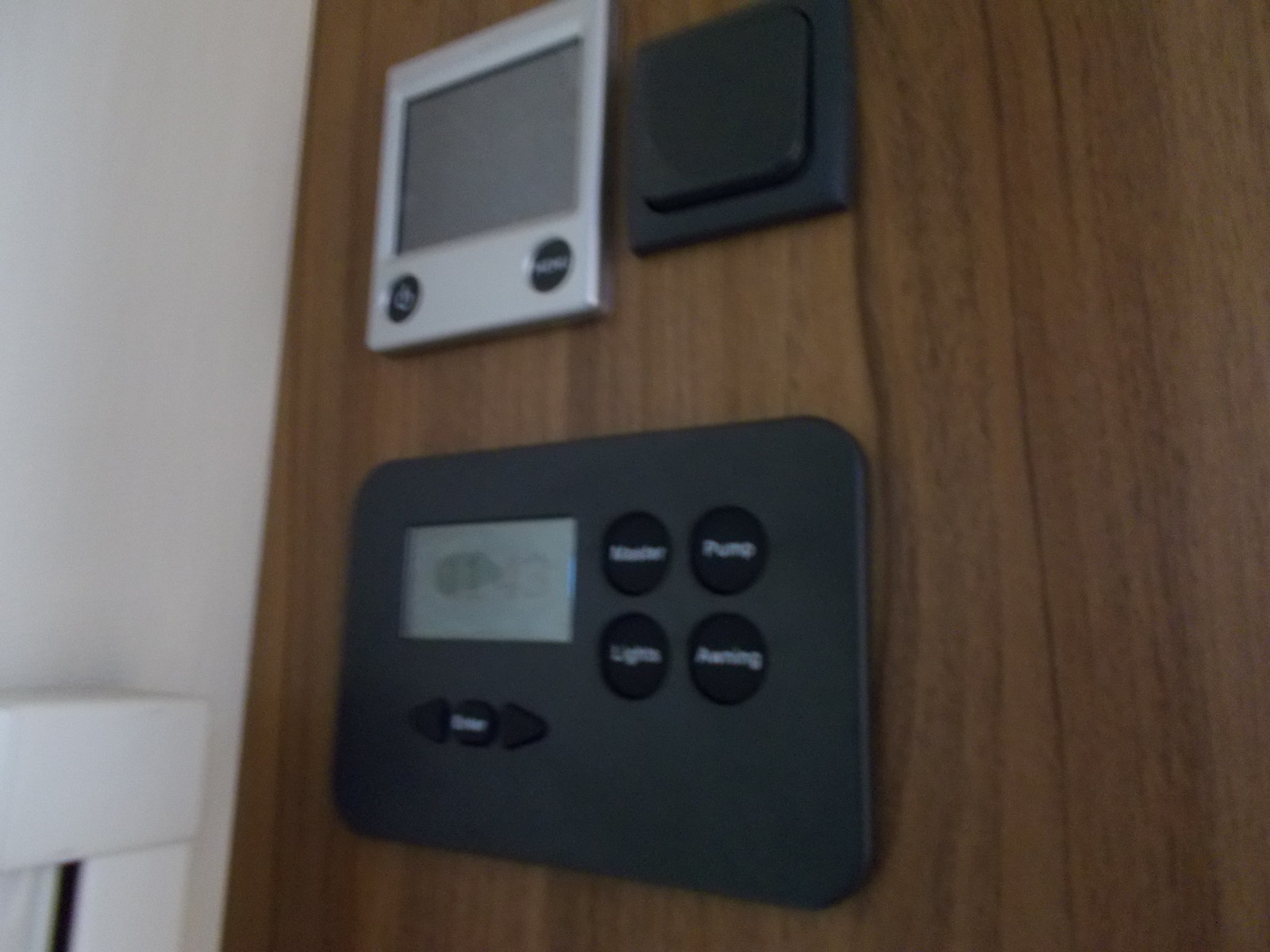The image depicts a set of three control panels mounted on a wooden wall, presented in a somewhat blurry photograph that obscures some of the finer details. The lower control panel is black and square-shaped, featuring an LED readout in the upper left corner. The background of the LED screen is gray, with black text displaying the numbers "1143." This panel includes several buttons, and while most labels are illegible due to the blurriness, two buttons are discernible, labeled "Pump" and "Lights."

Above this, there are two more control panels. The one on the left is silver and equipped with its own LED readout screen. Below this screen, there are two buttons, one situated on the left and the other on the right, though their labels remain unreadable in the image. The final panel to the right is an ambiguous, featureless black panel, which might be a control panel or possibly a speaker, but the blurriness of the photo leaves this unclear.

Overall, this setup of control panels is integrated into a wooden panel wall, presenting a somewhat modern though slightly indiscernible control interface.